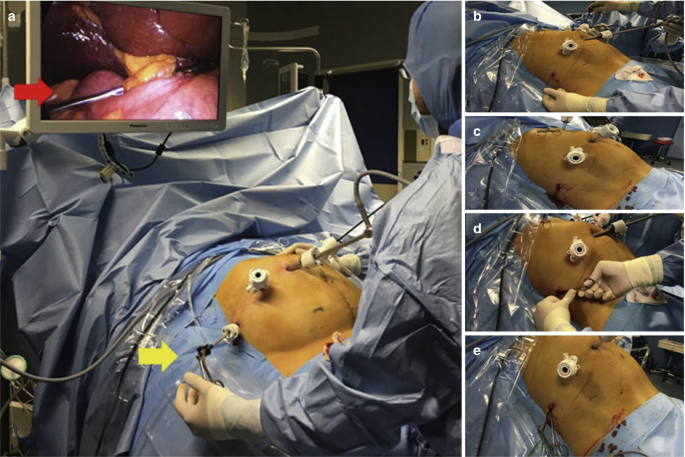The detailed photo montage depicts a robotic-assisted laparoscopic surgery procedure in a dimly lit operating room. Dominating the montage is a large central image labeled with a white lowercase "a" in the top left corner. In this primary photo, a doctor in surgical scrubs is attending to a patient whose body is mostly shielded by blue surgical sheets, leaving only the swollen abdomen visible, suggesting a possible special condition such as pregnancy. The patient's stomach is adorned with several small white tubes, approximately five, each serving as portals for metallic instruments, including forceps. A TV screen in front of the doctor displays the internal view, showing red and yellow hues illustrating the surgical actions. A red arrow points to this screen, while a yellow arrow points to the manual actions of the doctor. To the right of the main image, there are four smaller, equally distributed photos labeled "b," "c," "d," and "e," depicting various stages and angles of the procedure, further documenting the intricate steps involved.